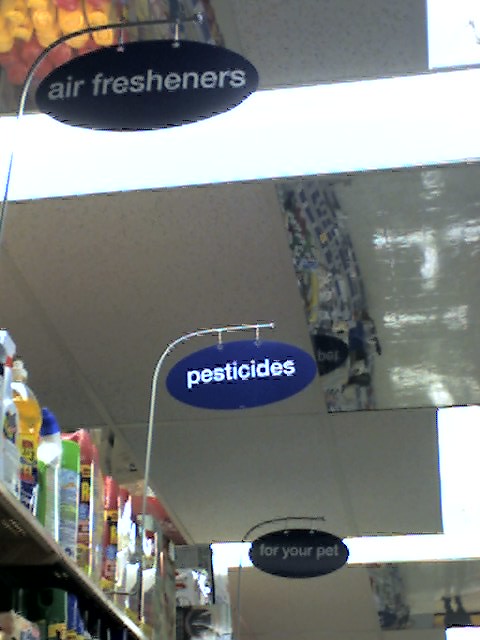This grainy, blurred photograph captures the interior of a store. The viewpoint extends from closest to the top of the image downwards and into the distance. On the left side, transitioning towards the center, there is a noticeable shelf stocked with what appears to be an assortment of bug sprays. Above this shelf, a blue oval sign with white text prominently reads "Pesticides". Nearby, another sign indicates "Air Fresheners" over an adjacent shelf. Towards the back, in a darker, grainier part of the image, a sign is discern visible, labeled "For Your Pet."

The ceiling of the store features a standard white drop ceiling commonly seen in many retail establishments. A vertical mirror is mounted on the ceiling, reflecting the shelves below it. Additionally, in the lower right corner of the photograph, another mirror can be seen, capturing the reflection of a shopper's foot and legs.